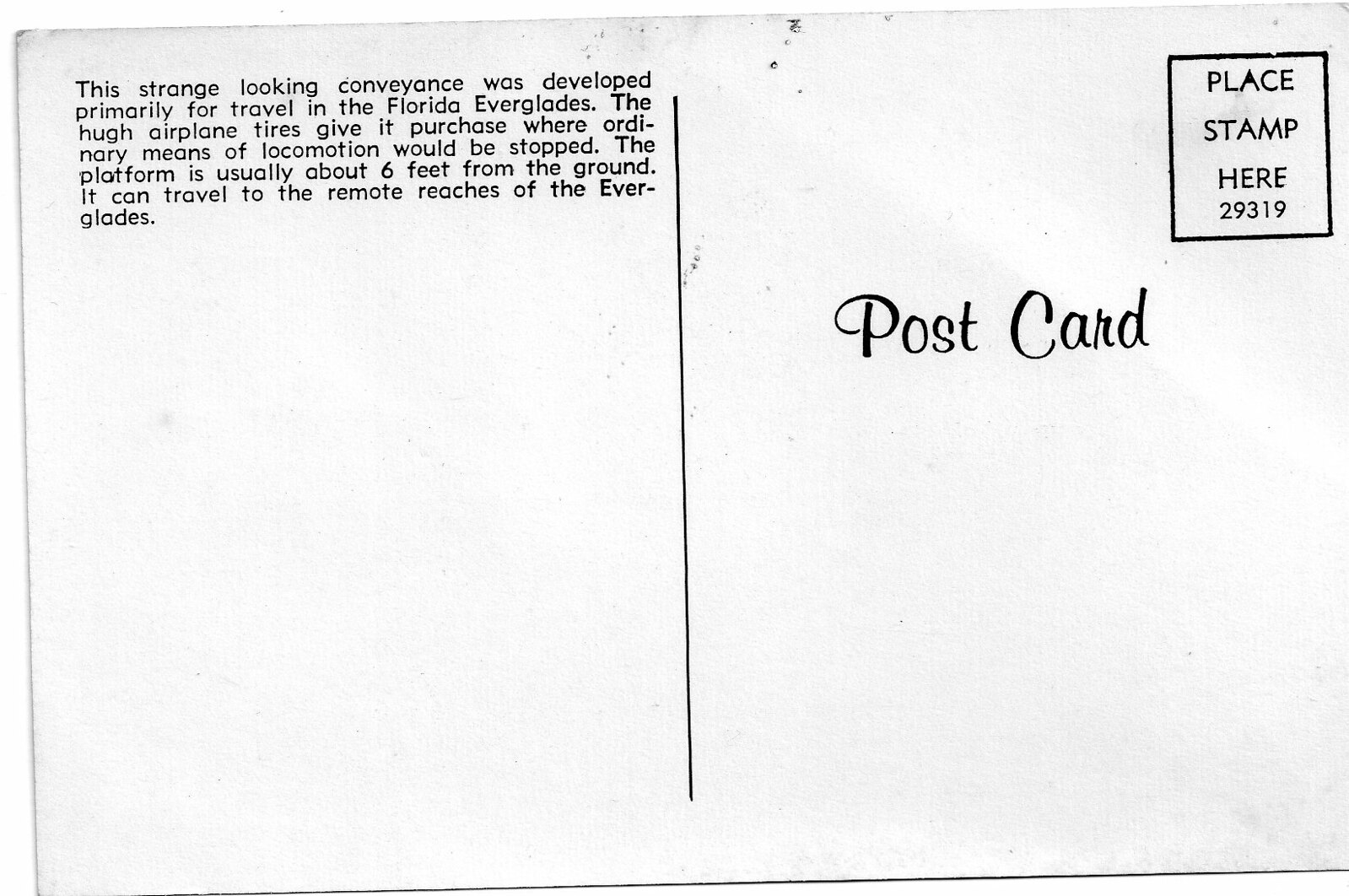This image showcases the back of a black-and-white postcard. In the top left corner, black text describes a unique vehicle designed for navigating the Florida Everglades: "This strange-looking conveyance was developed primarily for travel in the Florida Everglades. The huge airplane tires give it purchase where ordinary means of locomotion would be stopped. The platform is usually about six feet from the ground. It can travel to the remote reaches of the Everglades." A vertical black line approximately four inches long runs down the center of the card, dividing it. On the right side, "Post Card" is written in cursive-like text in the middle. In the upper right corner, there is a marked rectangle for a stamp with the words "Place Stamp Here" and the number "29319." The postcard lacks any stamp, image, or additional decoration.